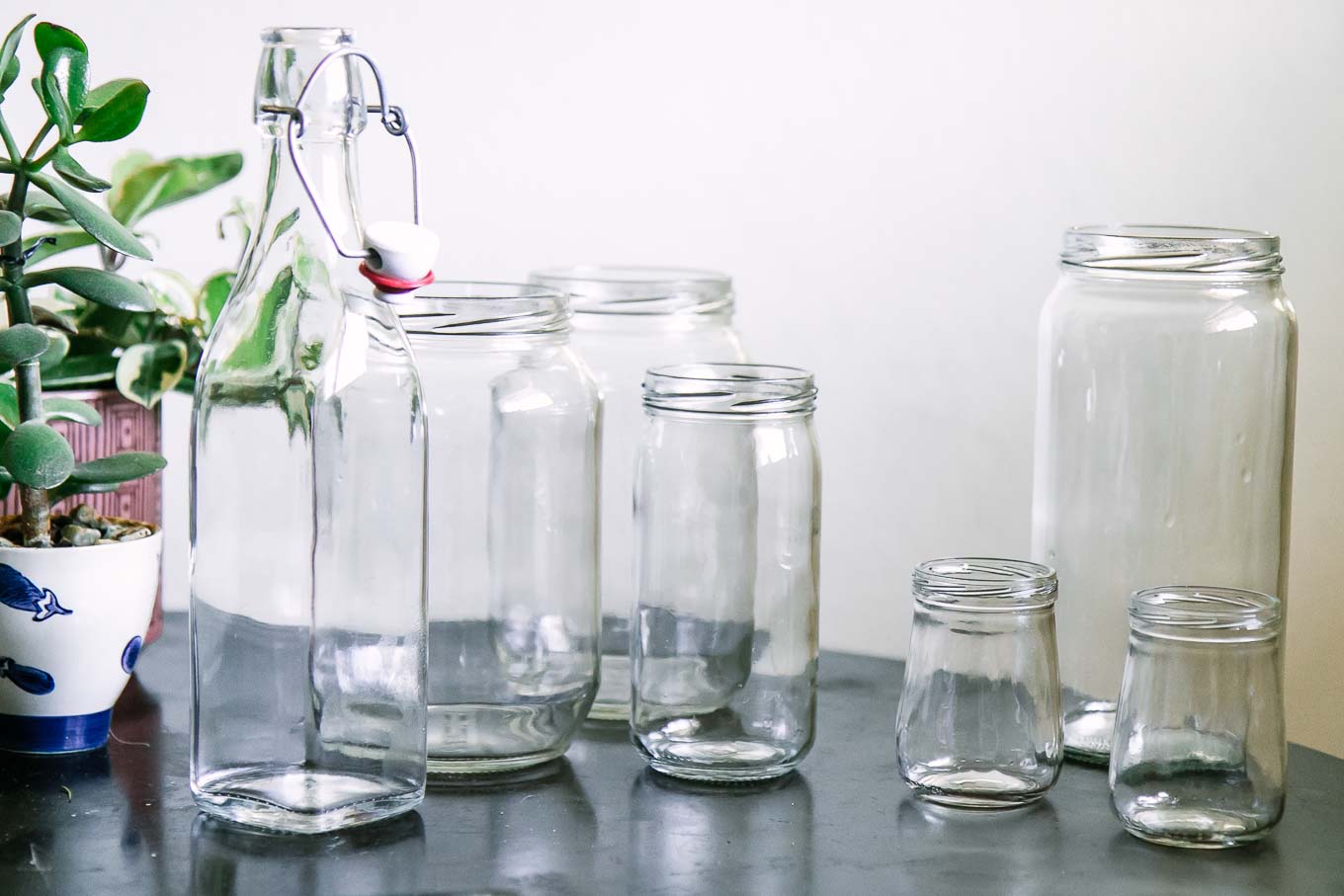This photograph showcases a neatly arranged assortment of clear glass jars and a single unique bottle, all sitting on a dark-gray countertop. The collection includes one tall, square bottle with a ceramic stoppered lid secured by a red rubber gasket and wire frame, ideal for storing liquids like vinegar or olive oil. The rest are plain, empty glass jars of varying shapes and sizes: two quart-sized jars, a narrow jar possibly for jam, two short jars that flare out at the bottom like mustard jars, and a taller, more squared jar behind them. To the far left, a charming jade plant is potted in a small, white and blue-glazed ceramic sake cup adorned with images resembling eggplants. Behind it, another plant with variegated leaves sits in a reddish-pink ceramic pot. The backdrop is a plain white wall, emphasizing the clean and organized arrangement of jars and plant life on the countertop.